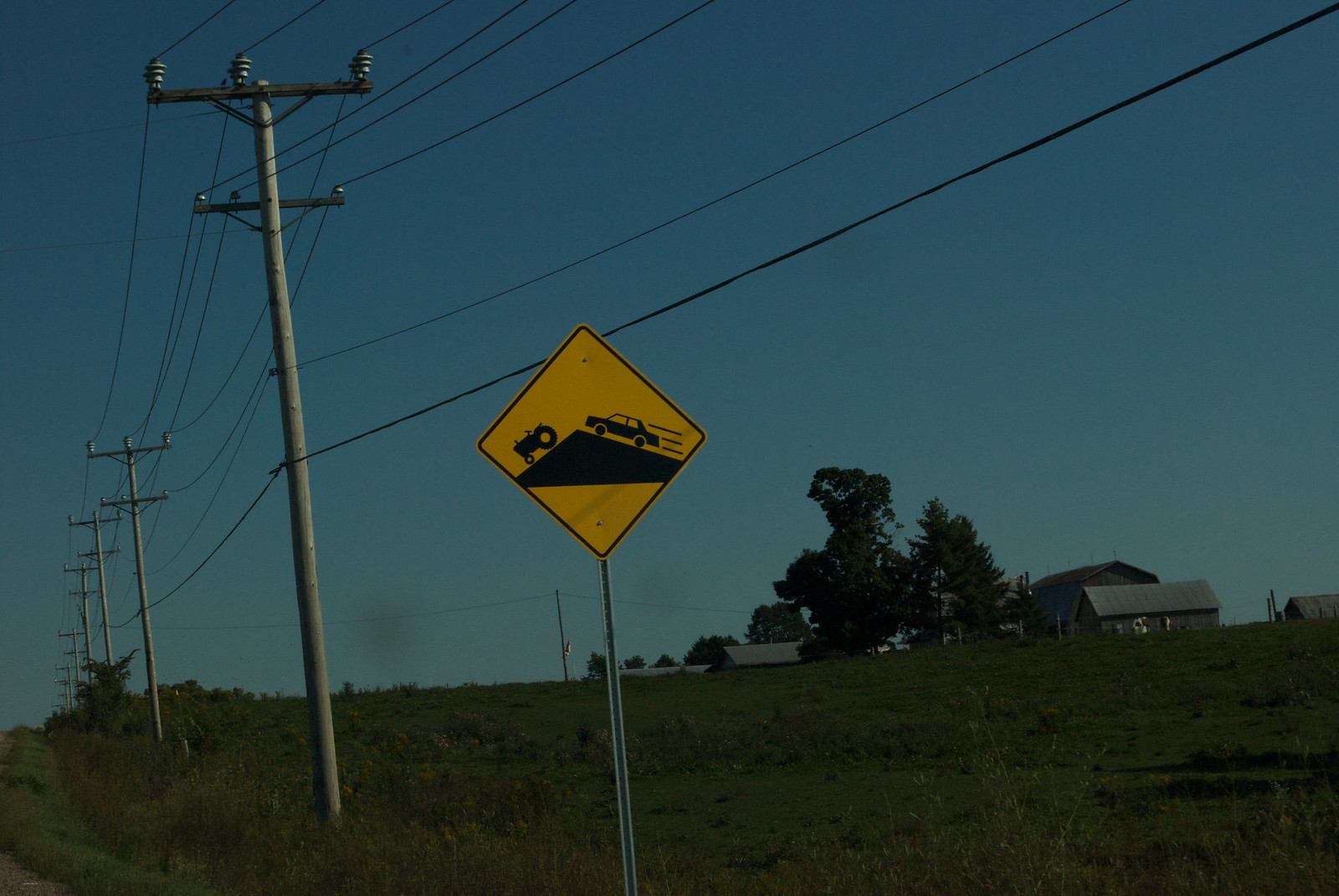The photograph captures a quintessential rural scene, set beneath a strikingly bright blue sky. Dominating the foreground is a distinctive yellow traffic sign mounted on a gray metal post. The sign features a black triangle depicting a car cresting a hill on the right side and a tractor descending the other side, clearly warning drivers of the potential for slow-moving vehicles on hilly terrain. Stretching across the landscape are wooden utility poles strung with numerous electrical and telephone lines, accentuating the rustic nature of the setting.

In the distance, a sprawling farmstead comes into view, complete with a farmhouse, a barn, and several smaller outbuildings. The area appears remote and agricultural, with a field in the foreground that seems to be filled with untended grasses and possibly weeds. Towering trees line the horizon, complementing the farm structures dispersed throughout the scene. The overall composition suggests a serene countryside setting where modern utilities meet traditional farming life, with the tilted angle of the camera adding a dynamic touch to the landscape.